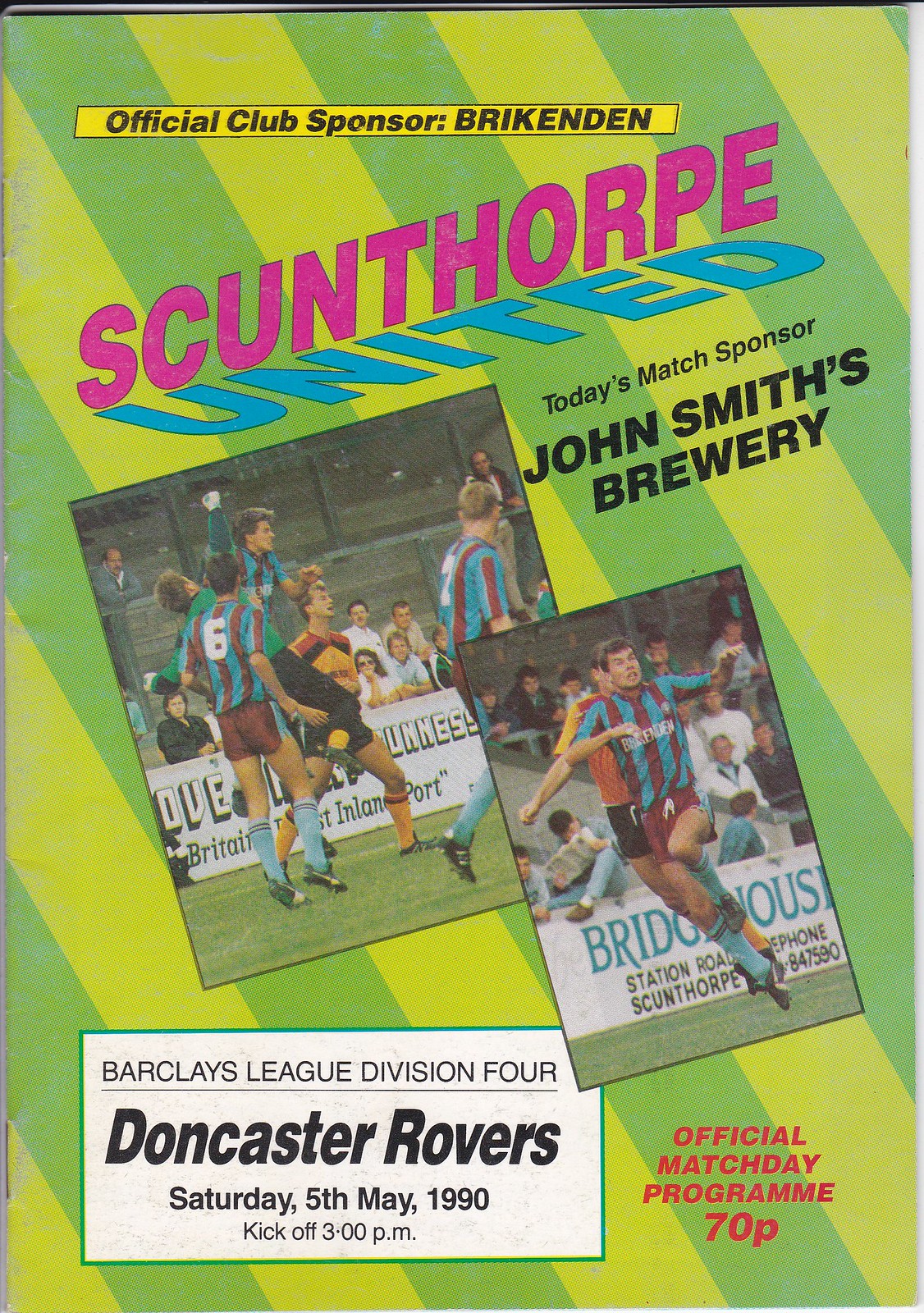The image is a vibrant and detailed cover for a soccer club's official match day program. The background features horizontally slanted stripes in various shades of yellow and green. At the top, a prominent yellow rectangle bears the text "Official Club Sponsor Bric-a-den" in small black font. Below this, "Scunthorpe United" is displayed, with "Scunthorpe" in purple and "United" in blue. The program highlights today's match sponsor, John Smith's Brewery.

Central to the design are two dynamic action photographs: one captures four players in mid-play with spectators watching, while another, superimposed over the first, focuses on a single player in full gallop, either chasing or having just kicked a ball. At the bottom, detailed match information appears: "Barclays League Division 4, Doncaster Rovers, Saturday 5th May 1990, Kickoff 3pm." In the bottom right corner, the price "Official Match Day Program 70p" is displayed in red. The overall color scheme encompasses vibrant yellow, green, purple, black, and white tones.